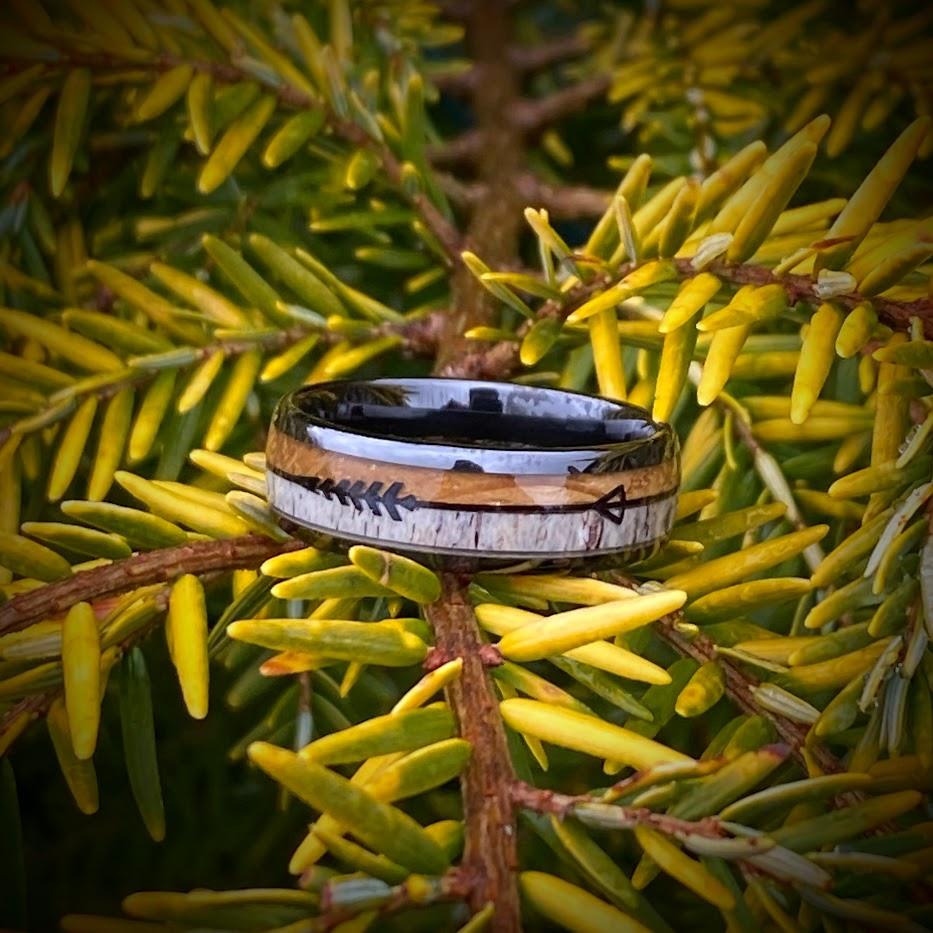A close-up image of a nature scene features predominantly green and yellow leaves with a thin, somewhat pointed shape resembling pine needles. The leaves are interspersed among brown branches and twigs. Amidst the foliage, there's a peculiar ring-like object resting upright on the branches. The ring has several distinct sections: the top is metallic and black, followed by brown, then another black stripe, gray, and finally black at its base. Although the image is closely zoomed in, a subtle, diffused light illuminates the scene without revealing its source.